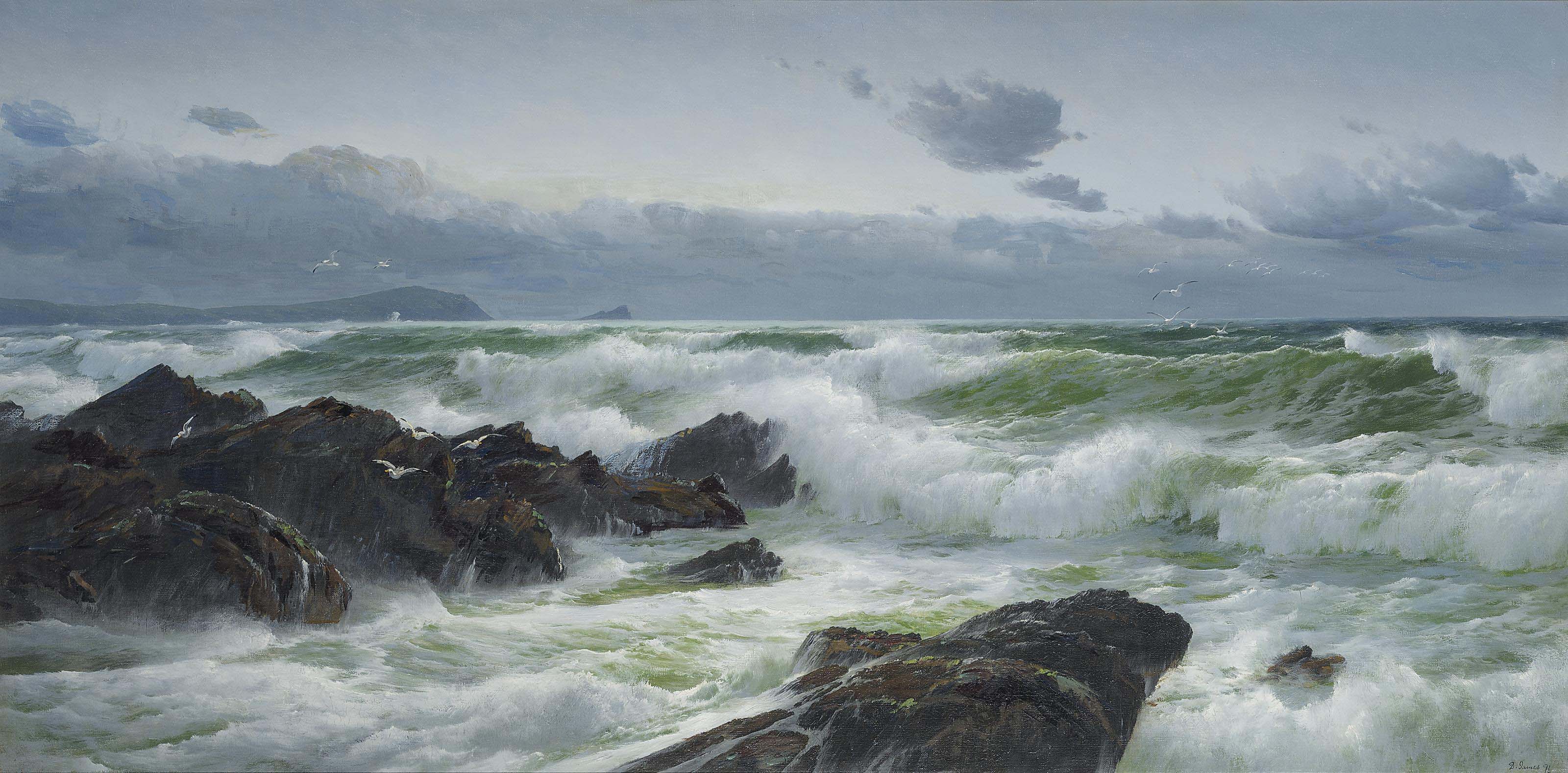The image is a hyper-realistic painting depicting a wild and ferocious ocean scene, almost photographic in its detail. The central focus is on large, powerful waves crashing against jagged, dark brownish-gray rocks that rise dramatically in the foreground. The ocean water exhibits a striking palette of navy blue, olive green, and bright, glassy green, with the waves crested in white. The intensity of the waves is palpable, as they surge and break into frothy foam against the craggy rock formations. 

Above, an overcast dusky gray sky dominates the scene, with clouds floating lazily and concentrated mostly towards the bottom part of the sky, giving a sense of depth and moodiness. To the far left, a slight hill or the beginning of a mountain is silhouetted against the horizon. The predominant colors of the scene—gray, white, green, and brown—contribute to an overall neutral and dramatic atmosphere, characteristic of a stormy, dusk-lit ocean. The painting captures the raw power and beauty of nature in exquisite detail.